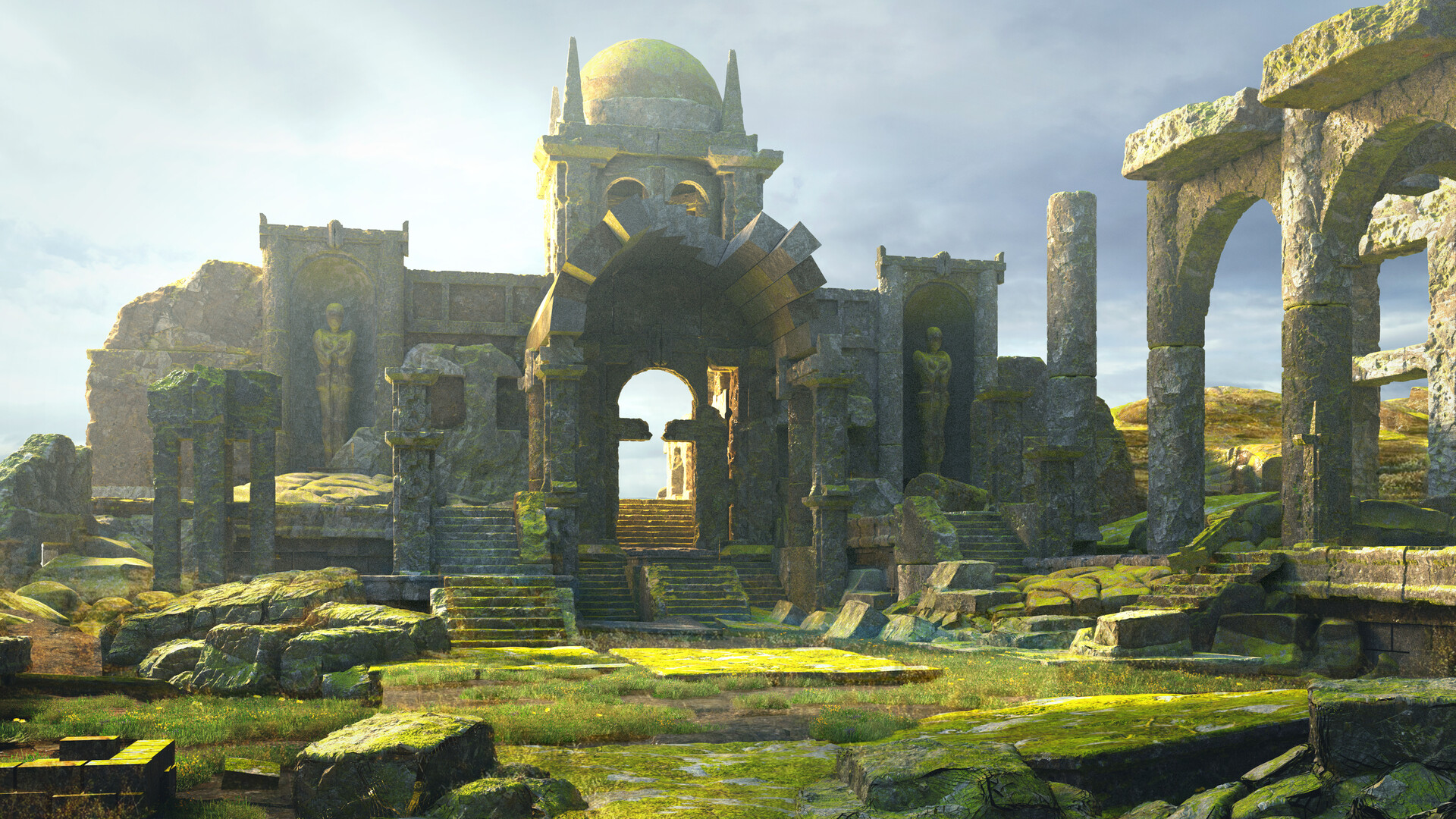The image depicts ancient ruins, potentially a screenshot from a video game or an AI-generated picture. The scene showcases a dilapidated temple or village entrance with significant architectural features. Dominating the image are two towering statues with arms crossed on their chests, flanking a grand stone archway topped with a dome. This archway leads into what was once a courtyard, now overrun with grass and moss. The ruins are primarily constructed of stone, though much of the original structure has crumbled, revealing a clear view through the arch to the surrounding landscape, which includes lush green hills and scattered trees. The sky is slightly foggy with some clouds, indicating daytime. The overall atmosphere evokes a sense of ancient, once-majestic beauty now reclaimed by nature.